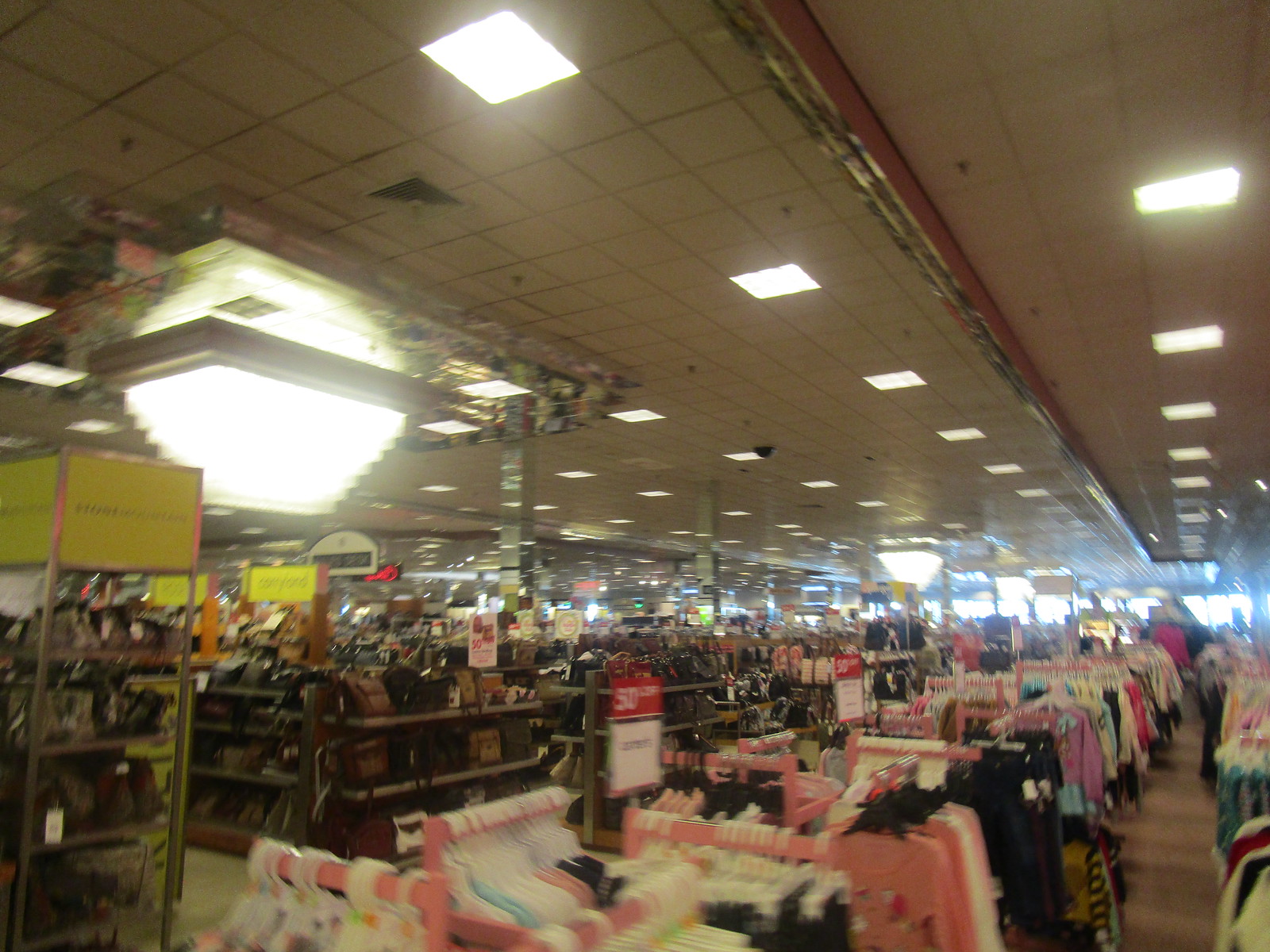A bustling department store interior brimming with diverse apparel dominates the image. The photograph showcases an expansive retail space characterized by a multitude of clothing racks laden with a vast array of garments. The bottom right corner of the image reveals an assortment of racks displaying an eclectic mix of women's clothing, including long-sleeved shirts, coats, and pants in a kaleidoscope of colors such as black, pink, purple, blue, and yellow. Prominently, some racks feature signs announcing a 50% off discount in bold red lettering.

On the left side of the image, additional racks appear to hold various leather goods, possibly purses and shoes, enhancing the store's assortment. The ceiling above is adorned with a grid of square lights interspersed with square white tile formations, providing a structured yet seamless illumination across the sprawling retail space.